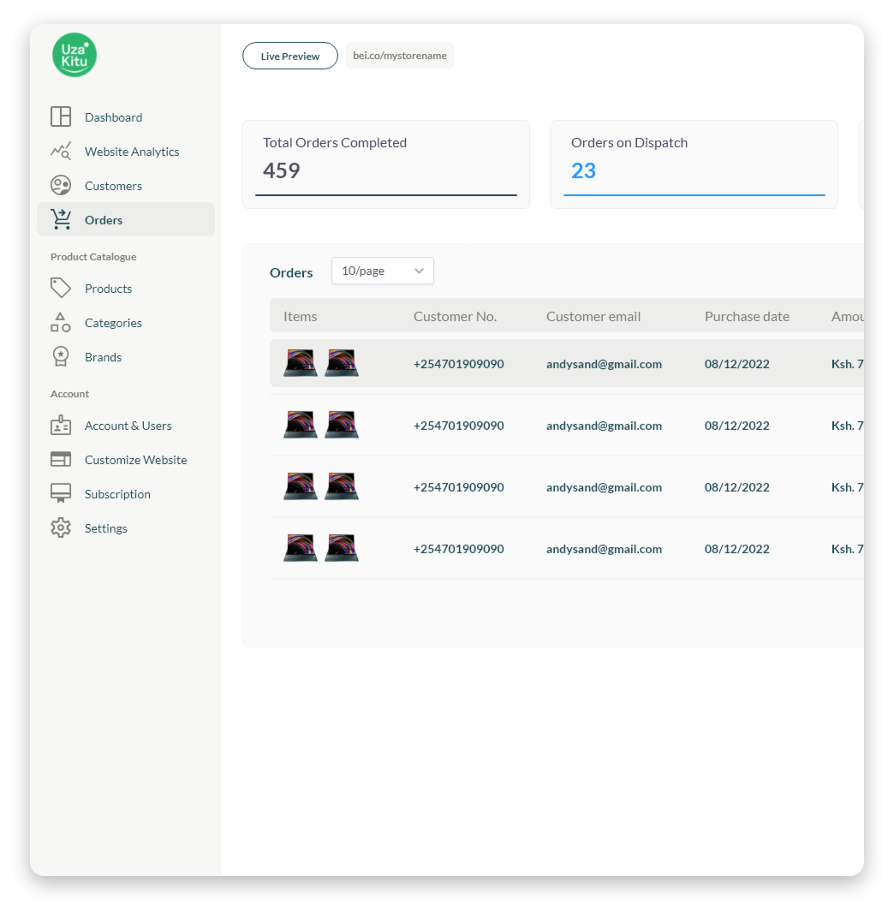A detailed screenshot of the "Uza Kitu" application interface, captured on a user-friendly, light gray background. In the top left corner, a green circle with white font spells out "Uza Kitu" (U-Z-A K-I-T-U). 

The sidebar reveals a well-organized navigation menu with various sections and categories, each accompanied by distinct icons for intuitive understanding. The first category includes options for "Dashboard," "Website Analytics," "Customers," and "Orders." Below is the "Product Catalog" section, comprising "Products," "Categories," and "Brands." The final category is labeled "Account," featuring subsections: "Account and Users," "Customized Website," "Subscription," and "Settings."

On the main content pane with a white background, predominantly black or blue text is displayed. At the top, a conspicuous button labeled "Live Preview" is outlined with dark blue, matching its font color. Adjacent to this, a light gray box shows the URL "BEI.CO/my-store-name." Further down, two light gray boxes summarize critical metrics: the left box displays "Total Orders Completed" in dark font, with a total of 459 orders underscored by a matching line. The right box indicates "Orders on Dispatch" with the figure 23 in light blue, paired with a similarly colored line.

Beneath these summary boxes is another labeled "Orders" in blue font, alongside a dropdown menu for adjusting the number of orders displayed per page, currently set to 10. The subsequent table lists all individual orders, providing a comprehensive overview of the order status and details.